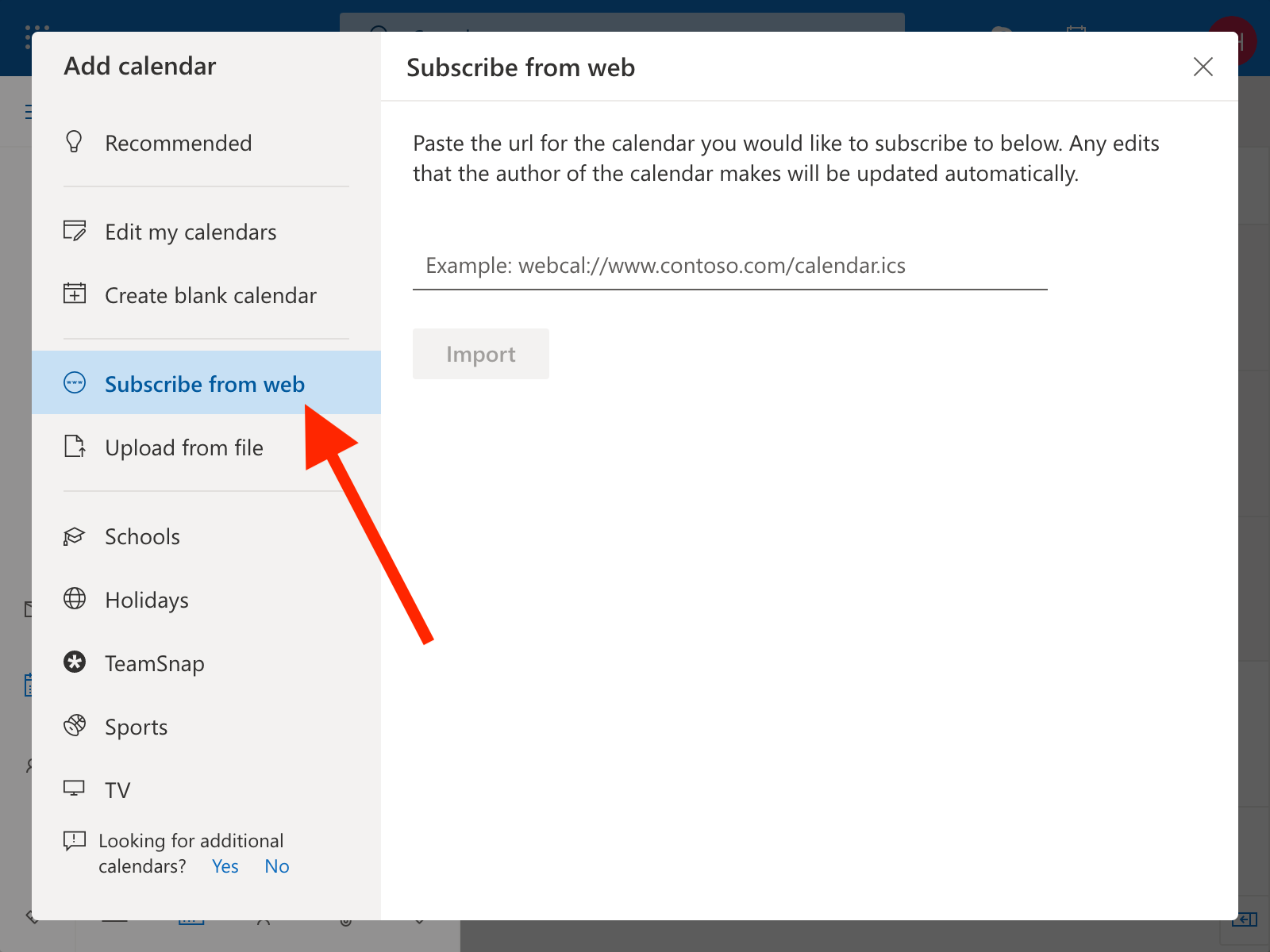In this image, we see the "Add Calendar" menu from a calendar application, likely Google Calendar, as it includes familiar interface elements. The highlighted setting, indicated by a large red arrow, points to the "Subscribe from web" option. This feature allows users to integrate a web-based calendar into their existing calendar setup by entering a specific URL. 

Additionally, the menu presents various options for managing calendars, such as editing existing ones, creating new blank calendars, and uploading calendars from a file. Users can also customize their calendar views to focus on specific events like school days, holidays, or sports schedules (such as those managed by TeamSnap). At the bottom of the menu, there is an option labeled "Looking for additional calendars," which can be toggled with a yes or no response, suggesting further customization features.

The overall layout demonstrates the multitude of ways users can personalize their calendar experience, catering to different needs and preferences.